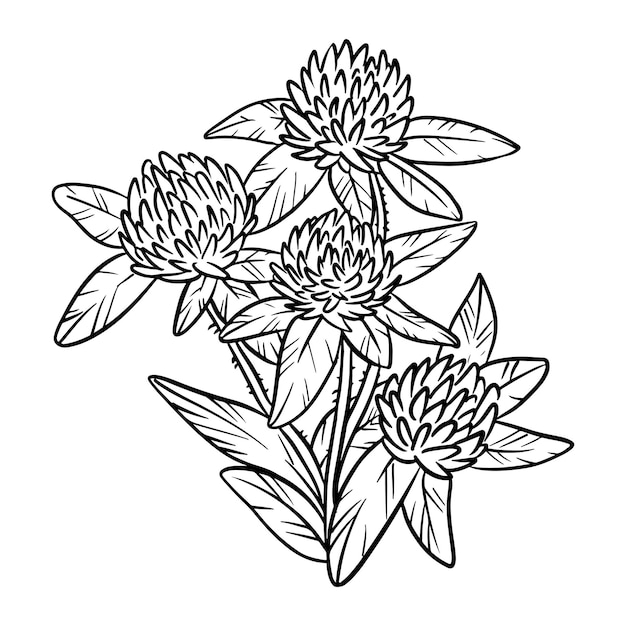This is a black and white clip art style drawing, reminiscent of an illustration you'd find in a coloring book, featuring a clump of four flower buds. The flowers closely resemble those of a clover plant, displaying the characteristic pom-pom heads of red, crimson, or white clover. Each bud is thick and packed with tightly clustered petals, giving a very dense appearance. The flowers are well-defined and detailed, with three prominently connected to stems. Leaves are intricately drawn with detailed vein patterns, showing a central vein with cross veins extending outwards. These leaves are longer with a somewhat pointed tip, closely bunching around the flower bases. A fourth flower is partially hidden towards the bottom, with its stem not visible, and additional leaves are depicted at the base of the clump. The entire drawing stands out against a stark white background, highlighting the careful black line details in the image.